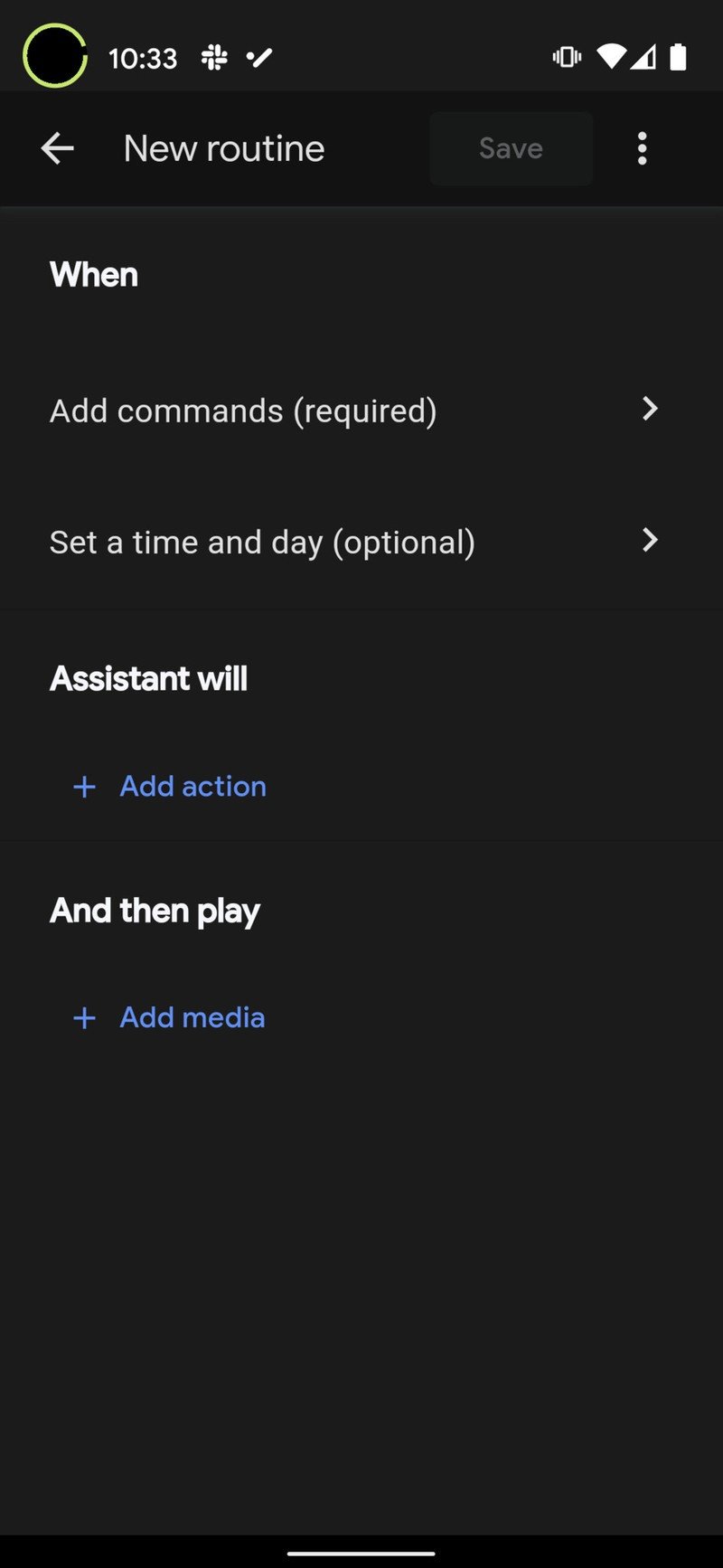The image is a screenshot taken from a mobile device displaying a user interface for setting up routines. The screen features a black background. At the top of the screen, on the right side, there are icons for battery life and Wi-Fi signal strength. On the left side, the current time is shown as 10:33, next to a green circle. Below this, there is a heading labeled "New Routine" with a back arrow to its left, and on the right, options to "Save" the routine and a menu represented by three white dots.

Under this heading, the word "When" is displayed in white text, followed by the instruction "Add commands (required). Set a time and day (optional)." Written in bold white text directly below this, the section "Assistant will" appears, accompanied by a blue button labeled "Add action." Further down, the text "And then play" is written in white, with another blue button labeled "Add media" beneath it.